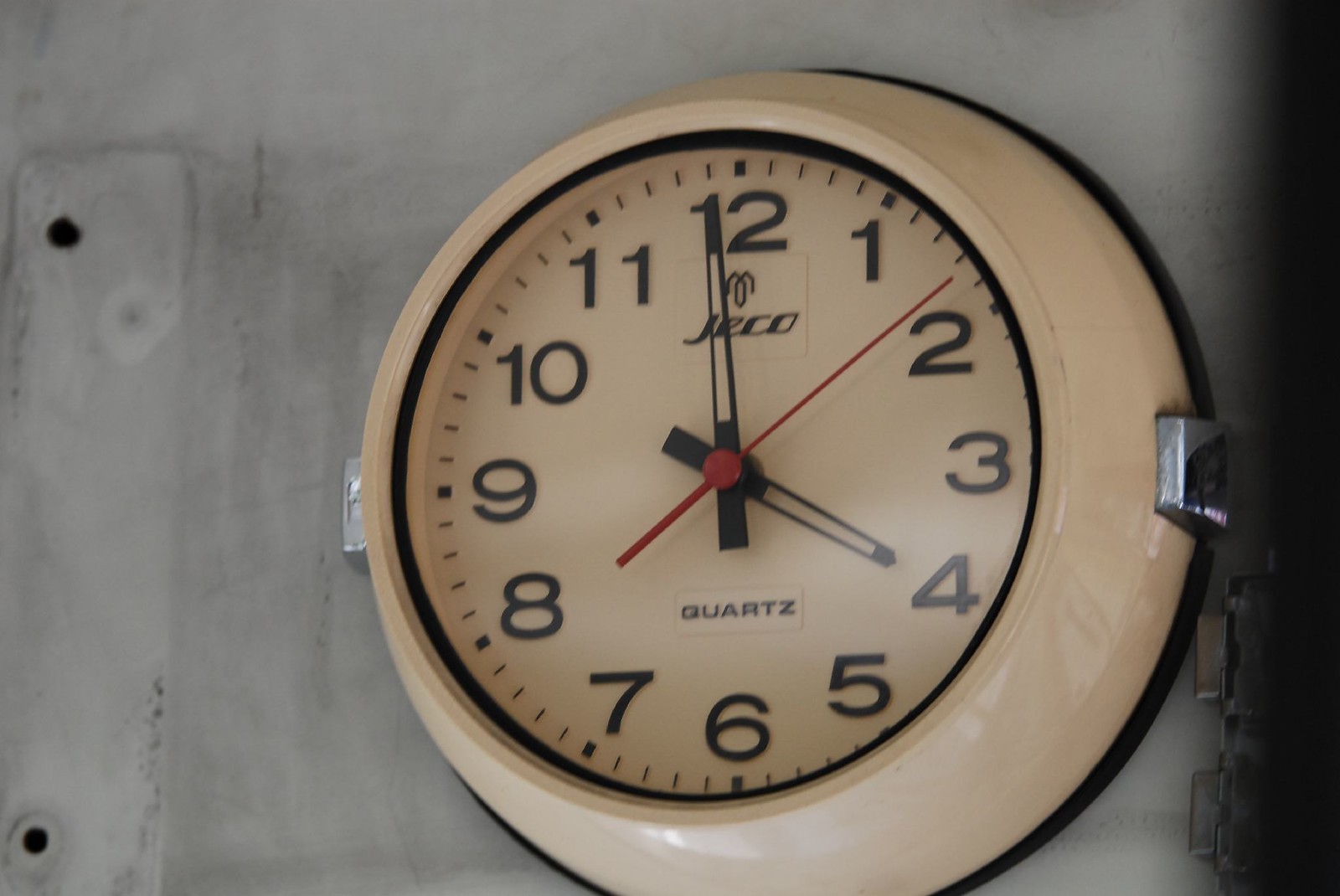A beige wall clock, prominently positioned in the center of the image and extending slightly towards the right, displays the time as 4:00. The clock, resembling those commonly found in offices or schools, features black hour and minute hands, a red second hand, and black numbers. The face of the clock also bears the brand name "JECO" and the word "Quartz" beneath it. The wall behind the clock is gray and appears worn, with noticeable scratches and multiple small holes, suggesting the prior presence of a bracket or similar fixture. Additionally, there is a faint rectangular outline on the left side of the image. A subtle shadow falls on the right side of the clock, adding depth to the scene.